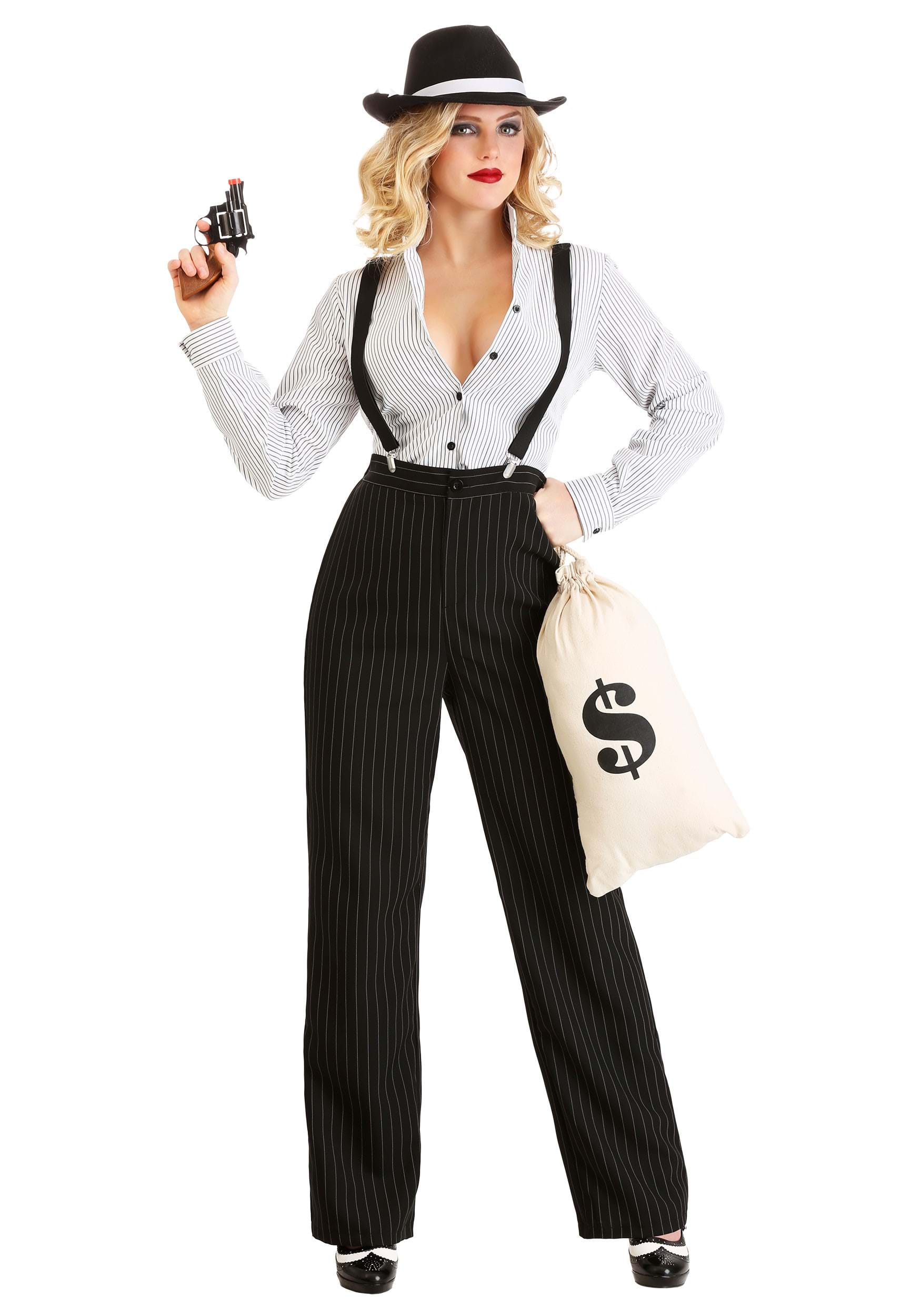The image showcases a woman dressed as a bank robber, likely for a Halloween costume. She has medium-length curly blonde hair and is adorned with striking red lipstick and heavy makeup. She is posed with a confident stance, her head cocked to the side. Her outfit features a black fedora with a white ribbon trim, a revealing black pinstripe button-down long-sleeve shirt with suspenders clipped onto her high-waisted black pinstripe pants. Her shirt is unbuttoned to mid-chest, exposing some cleavage. She wears black dress shoes with white accents. In her left hand, she holds a cream-colored burlap bag emblazoned with a dollar sign, indicating stolen money, and in her right hand, she brandishes a toy revolver aimed in the air. The background is stark white, devoid of any text or additional context.